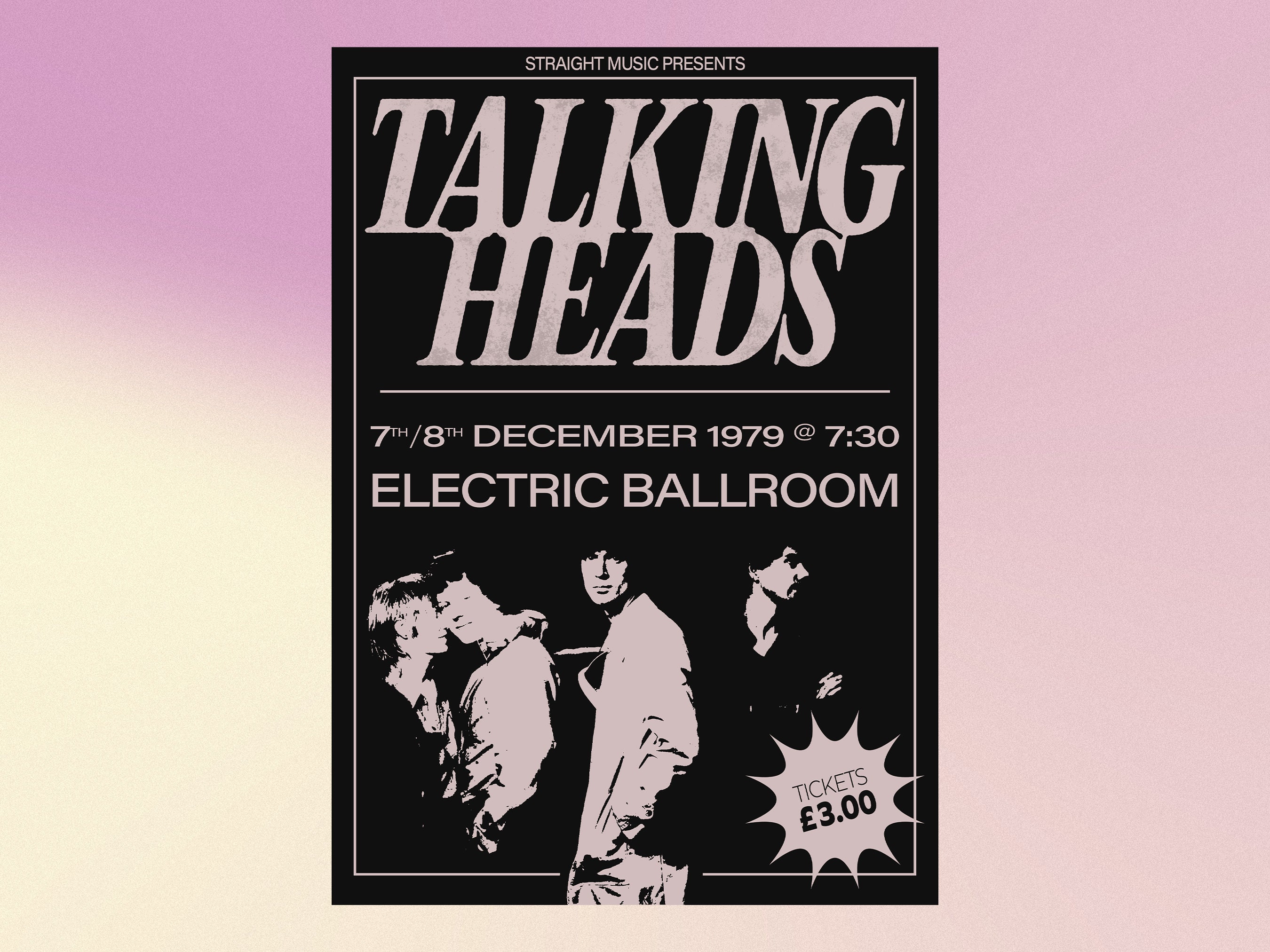This detailed image showcases a vintage poster advertising a Talking Heads concert presented by Straight Music, held on December 7th and 8th, 1979, at 7:30 PM at the Electric Ballroom. The poster is set against a striking background featuring a gradient of pinkish-purple hues that blend seamlessly into bright yellow and white tones, evoking the appearance of a sunset or sunrise. The dominant black poster is centrally positioned and has a white rectangular outline encasing the event details. At the top, "Straight Music Presents" is written in small white text, followed by bold, large white letters spelling out "Talking Heads." Below this title is a white line, under which the dates "7th-8th December 1979 at 7:30" are specified. Further down, "Electric Ballroom" is written in white. The lower section of the poster contains three black-and-white images which appear to be band members: two men embracing on the left, a stoic individual in a side profile facing us in the center, and a separate individual facing away on the right. In the bottom right corner, there's a pointed circular shape with the black text inside announcing "Tickets £3."